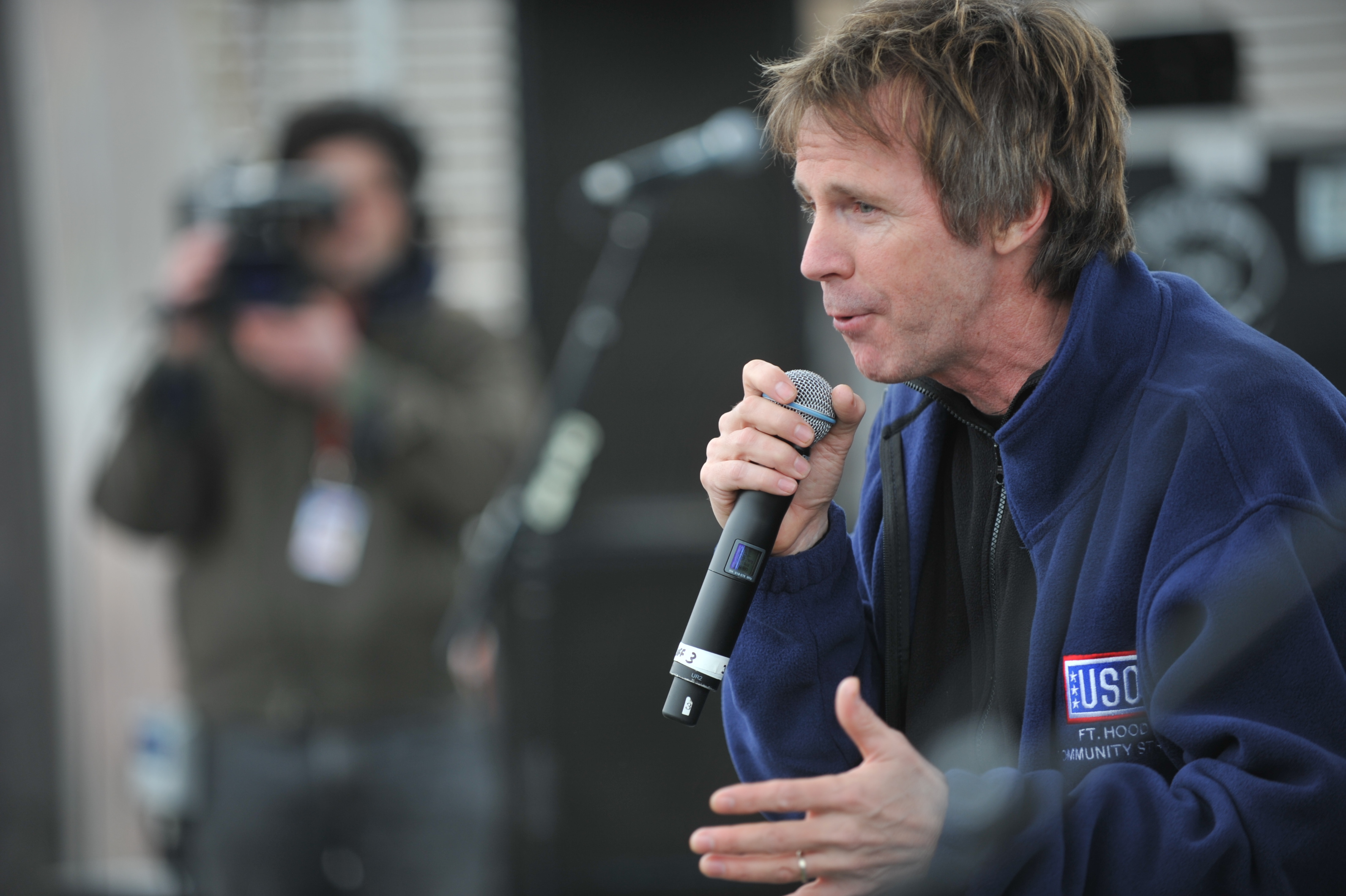In this brightly lit, well-focused photograph, a man is positioned on the right side of the image facing left, holding a black-handled microphone with a silver head in his right hand. He is attired in a navy blue fleece jacket embroidered with "USO Fort Hood" on the chest, layered over a black zip-up fleece. The man, light-skinned with short, dark blonde, somewhat shaggy hair, bears a resemblance to Dana Carvey. On his left ring finger, he wears a gold wedding band. The background is intentionally blurred, though it reveals a cameraman recording the scene.